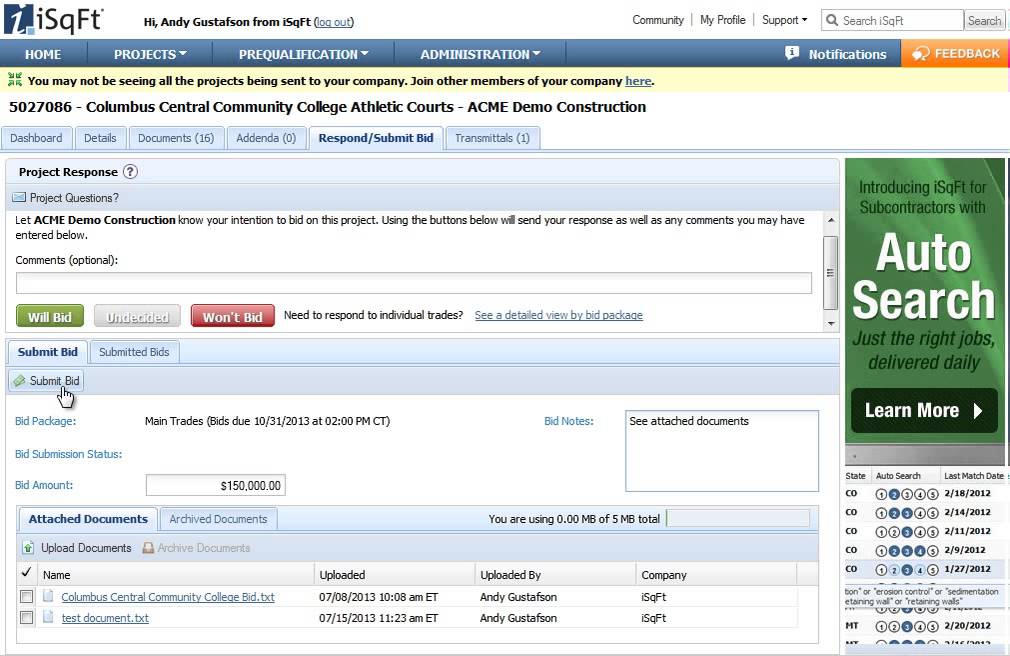Screenshot Description: Dashboard Overview for Bidding and Project Management

The screenshot depicts the dashboard interface of a project management and bidding platform, specifically showcasing details for Columbus Central Community College's athletic courts, managed by ACME Demo Construction. At the top, the system greets the user with "Hi, Andy," and notes that "Gustaf is home from I, square foot." The dashboard includes a navigation menu with options for "Home," "Projects," "Prequalifications," and "Administrations."

A critical message alerts users that they might not be seeing all projects sent to their company and encourages them to join other community members, offering a contact number for assistance. Several projects are listed, prominently featuring "Columbus Central Community College, Athletic Courts," with project details including different statuses like "Will Bid," "Undecided," "Won't Bid," and a button to "Submit Bid." The main trades involved are also noted.

Project details include: 
- Project Date: 2013
- Document Attachment: Test Document, 2013

On the right side, an advertisement occupies a portion of the screen. The dashboard also features sections for "Community," "My Profile," "Support," "Feedback," and "Notification." Given the interface's appearance and references to the year 2013, it has an older design, potentially indicative of a Windows program from that era.